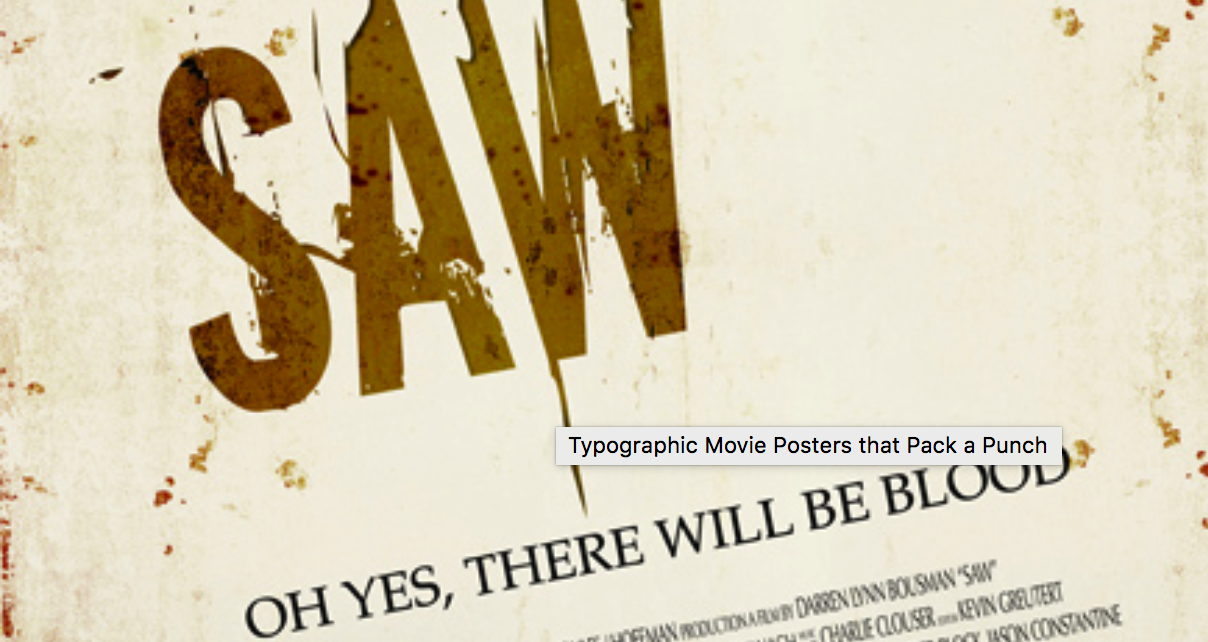This image is a close-up photograph of a movie poster for the horror film "SAW." Dominating the design, the title "SAW" appears in bold brown letters over a cream background, which features scattered brown and red stains, lending a gritty texture to the poster. Diagonally from left to right, the chilling tagline, "Oh yes, there will be blood," is prominently displayed, setting a grim tone. At the bottom, a white rectangular overlay contains the text, "Typographic movie posters that pack a punch," written in black. The poster also includes production credits naming Darren Lynn Bousman, Charlie Clouser, Kevin Greutert, and a partially visible name, Jason Constantine, against the characteristic off-white and stained backdrop. The stark and unsettling design effectively captures the essence of the "SAW" series.